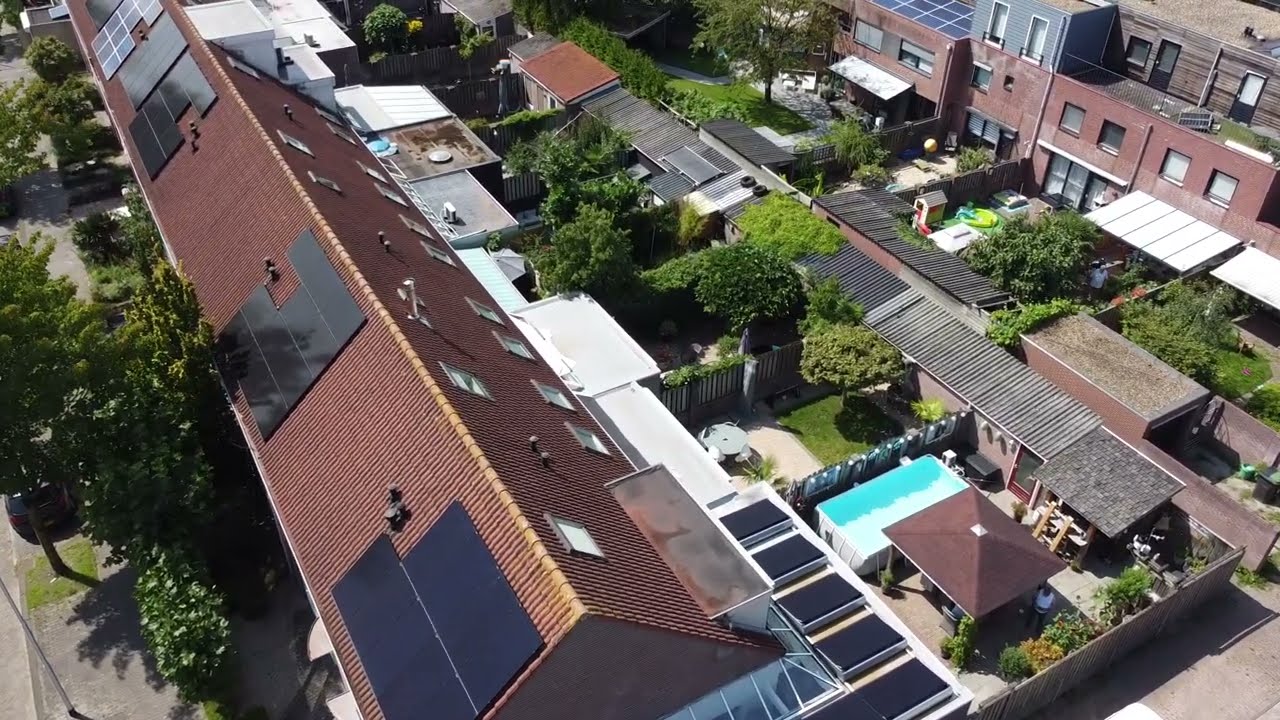Aerial drone shot of a densely-packed residential area, featuring rows of connected buildings with brown, triangular roofs. Approximately half of the roofs are outfitted with solar panels, while the others are not. Below, visible in their backyards, are small, fenced gardens, some with grass or trees. Notably, one house stands out with a sizable swimming pool in its yard. Between the two rows of buildings runs an alleyway, with additional greenery and trees lining the streets in front. There are no visible parking areas, only small sheds likely used for storage, further emphasizing the cluttered nature of the community.